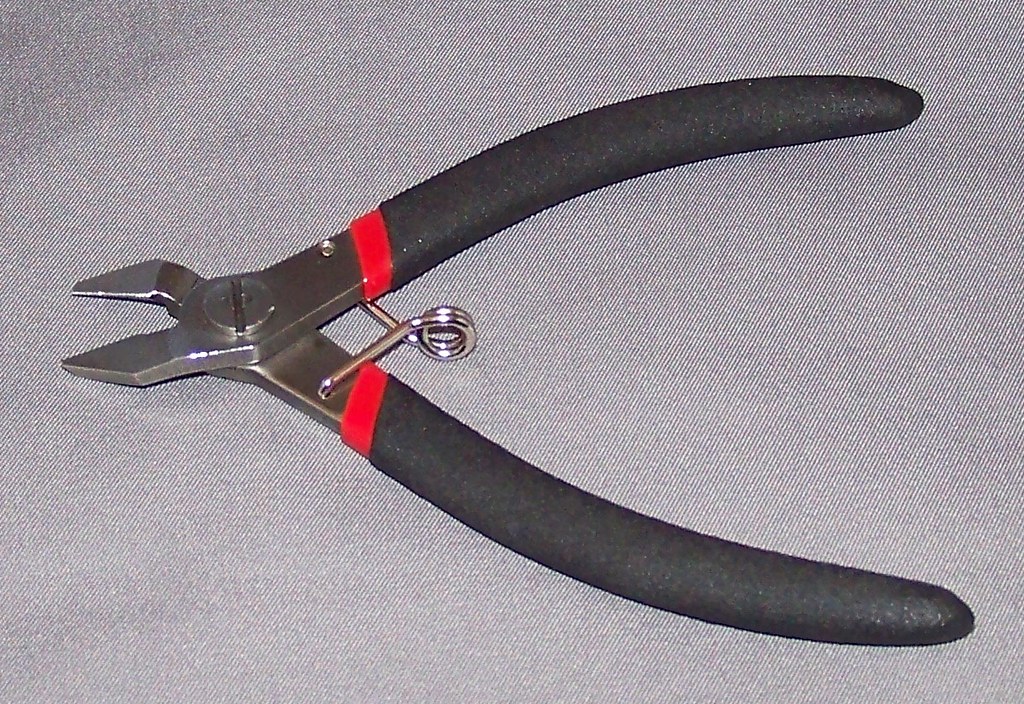The image features a pair of small, sharp wire cutters, commonly used for tasks such as jewelry making or cutting thin materials like wire or tin. The cutters have ergonomic black handles with a soft, comfortable grip, enhanced by a red band near the top for better handling. A silver coiled spring situated between the handles provides tension, ensuring the tool opens and closes smoothly. Additionally, a large, silver round screw with a line through it is visible, which tightens or loosens the tool's mechanisms. The sharp cutting edges meet to effectively cut materials when the handles are squeezed. The wire cutters are placed on a textured, gray fabric background, adding further visual detail to the image.